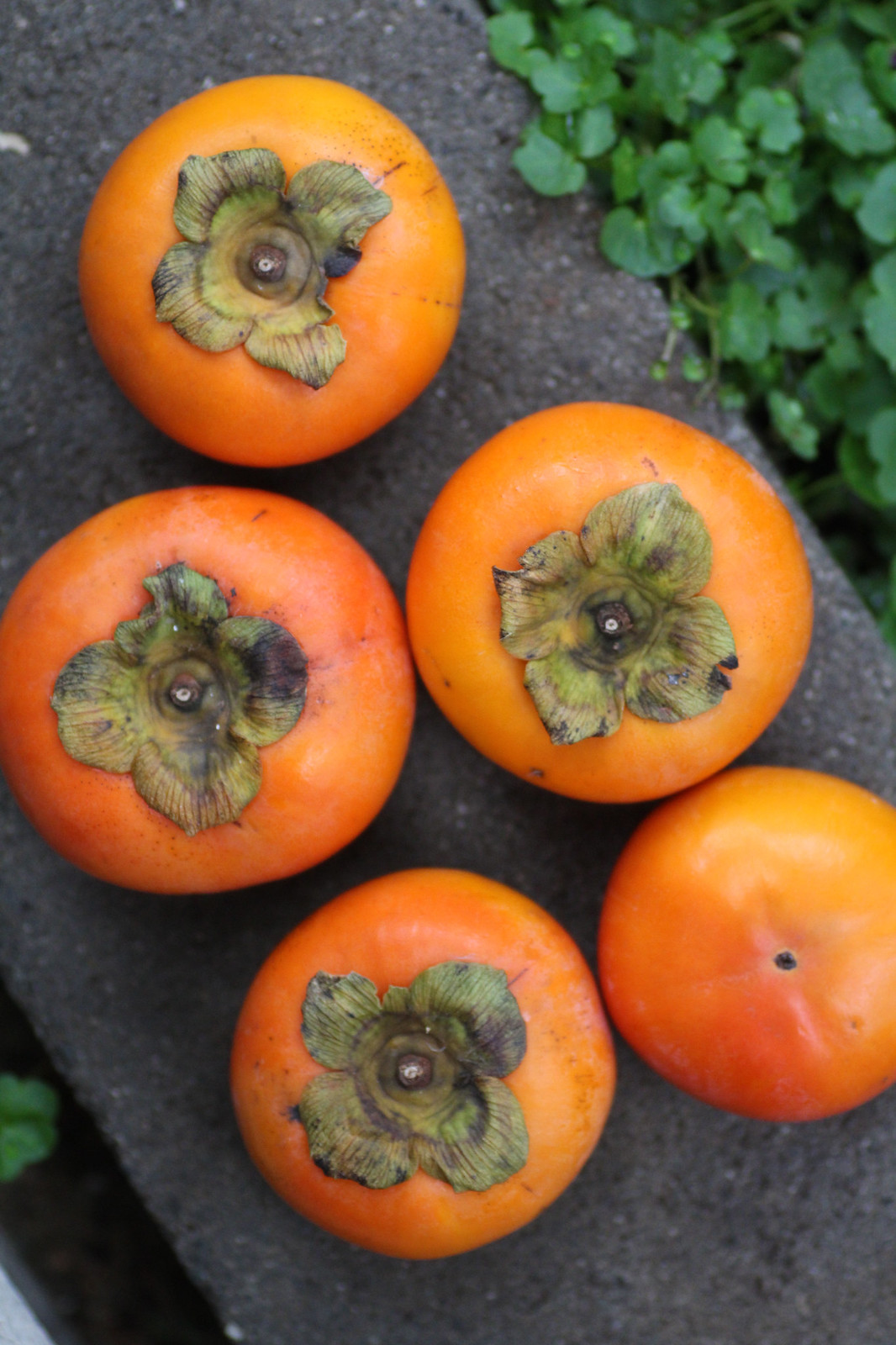In this bird's eye view photograph, five round, orange-colored fruits resembling persimmons are neatly lined up on a short, black stone ledge, possibly in a garden. Surrounding the scene, there are various green plants and leaves visible, hinting at an outdoor setting. Each fruit has a green stem and some small leaves on top, although one fruit appears to be either missing its stem or is upside down, showing a small brown spot instead. The stems and leaves look a bit dried and shriveled, yet the fruits themselves appear ripe and edible, with shades ranging from deep orange to slightly yellowish hues. The layout spans from the top left to the bottom right of the image, with a large fruit in the upper left corner, followed by two more in the middle, and two smaller ones at the bottom. Dirt on the fruits suggests they may have just been picked and haven’t been washed yet.